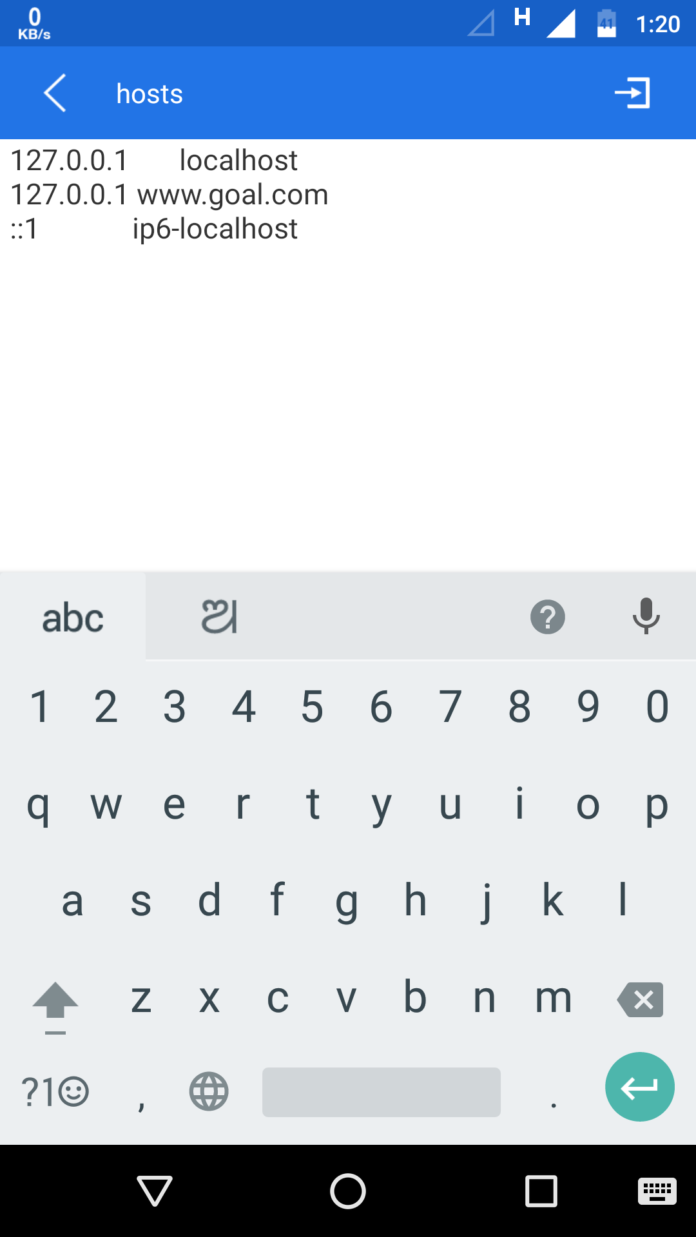This image, captured from a smartphone, showcases a screen displaying a text editor or terminal interface. In the upper-right corner, there are standard indicators including the time, battery level, and cell signal strength. The upper-left corner features a "0 kb" indicator, suggesting that there might be no active downloads at the moment. 

Prominently, a virtual keyboard is visible on the screen with a full set of numeric keys (1-0) and alphabetical letters, indicating that text input is being used. The interface appears to be a code editor or configuration file viewer. 

Three lines of text are displayed in the main area of the screen. 
The lines are as follows:
1. "127.0.0.1    localhost"
2. "127.0.0.1    www.goal.com"
3. "::1    ip6-localhost"

A blue bar labeled "hosts" is situated just below the status bar, identifying the file being edited as the hosts file, commonly used to map hostnames to IP addresses.

At the bottom, a black bar contains controls allowing for the minimization of the keyboard, reinforcing that the image is taken from a phone. The overall context suggests the user is modifying or viewing a system configuration file related to network settings.